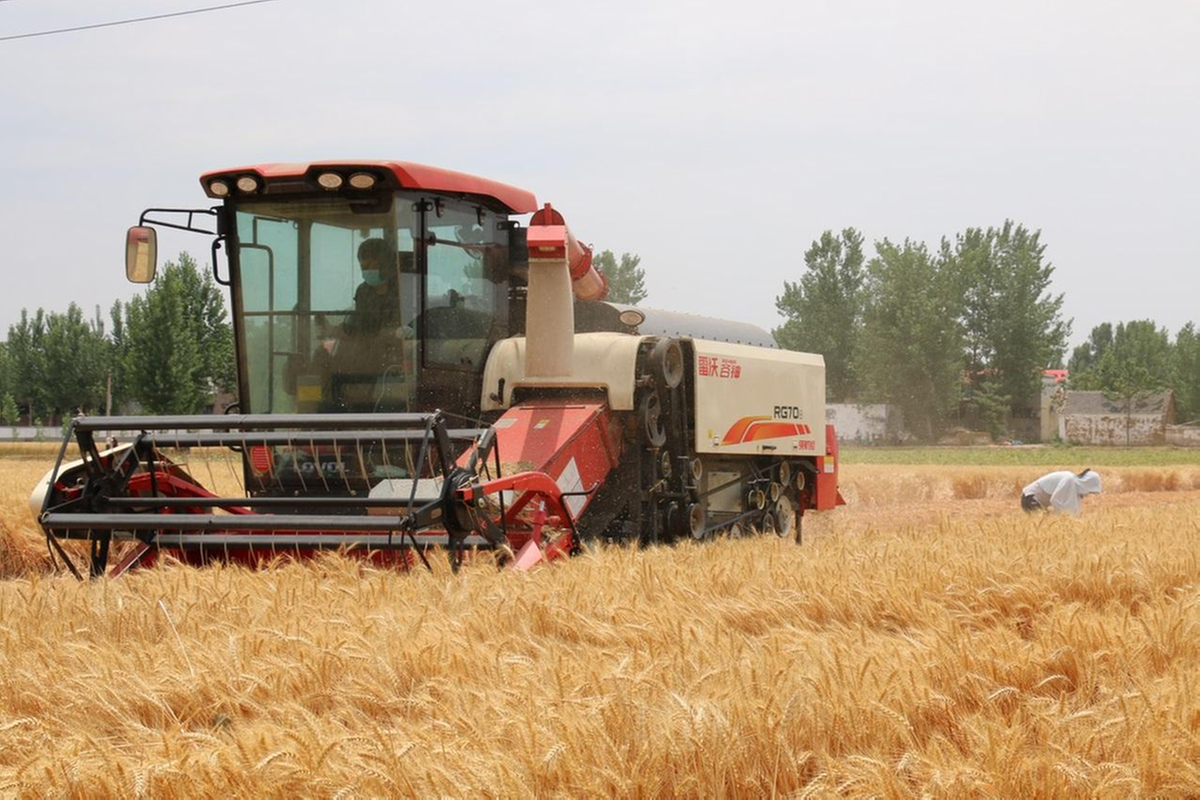The photograph captures an outdoor scene on a farm, featuring a large piece of farm machinery, likely a combine harvester, positioned slightly left of center in a sprawling field of golden wheat. The machine itself has a robust, rectangular structure painted in red and white, with a large cab at the front that has glass windows on multiple sides and is covered by a red metal roof. Inside the cab, a person can be seen operating the machine.

The side of the combine facing the camera displays an elaborate system of pulleys and gears exposed beneath a metal plate. A prominent red chute extends upward from the front part of the harvester, curving back into the main body of the machine, suggesting a mechanism for collecting or processing the harvested crop. In front of the combine, there's also a black reel likely used for cutting and gathering the wheat.

To the right of the combine in the field, another individual in a white hoodie is bent over, seemingly engaged in some manual task among the crops. This scene occurs under a gray, overcast sky, lending a hazy appearance to the day.

In the background, a line of green grass separates the wheat field from a cluster of white-framed buildings and trees, creating a picturesque backdrop to the farming activity. The overall ambiance of the image speaks to the labor and machinery involved in agricultural work.